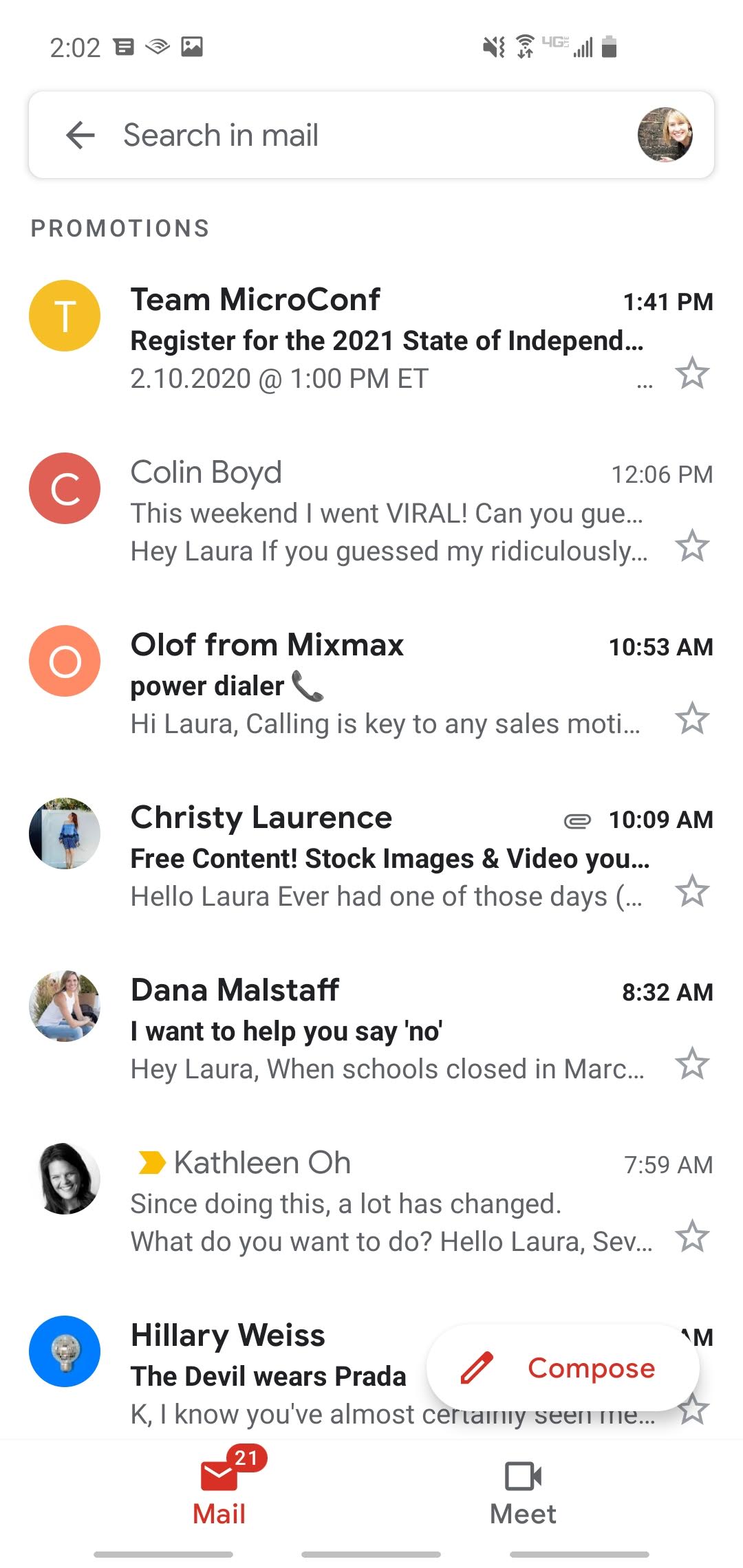In the upper left corner of the image, the time is displayed as 2:02. Below this, there is a large search bar with an arrow pointing left, labeled "search in mail" in the information box. On the right side of the image, there is a circular icon featuring a woman's face, and underneath this, the label "Promotions."

The first entry features the initial "T" in a yellow circle, followed by the name "Team MicroConf," and it was sent at 1:41 p.m. Below this, the initial "C" appears in a red circle, indicating a message from Colin Boyd sent at 12:06 p.m., with the subject line "This weekend, I went viral."

Next, there is a pink circle with the initial "O," indicating a message from Olof from Mixmax, sent at 10:53 a.m. Below, there is an image of a phone under the label "Power Dialer." 

Following this, there is another circular icon featuring the image of a woman standing against a white wall, representing Christy Lawrence. The corresponding message titled "Free content: stock images and video" was sent at 10:09 a.m.

Further down, an image of a woman in a white dress is visible beside the name Dana Maystaff. The associated message is titled "I want to help you say 'no'," with "no" in quotations. 

Finally, at the bottom, there is a blue circle beside the name Hilary Weiss, and the bolded text reads "The Devil Wears Prada." Positioned to the right of all these entries is the "Compose" button, depicted as a red pen inside a white circle.